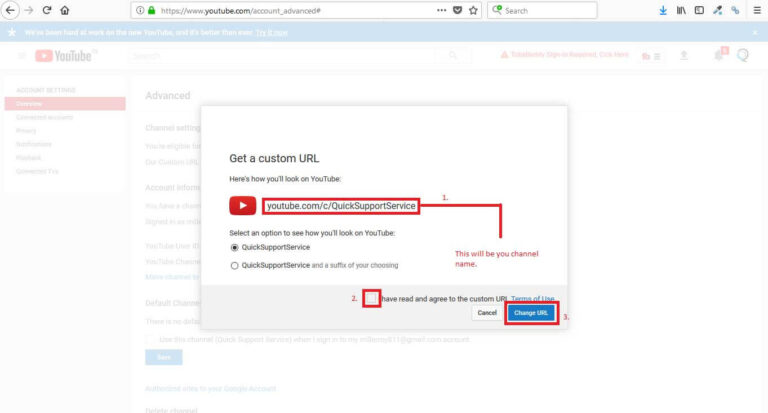The image showcases a web browser screen open to YouTube. In the top left corner is the URL "youtube.com," accompanied by a mini search bar to the right. Adjacent to these are six computer icons. The very top left corner features navigation buttons: a back button, a forward button, a refresh icon, and a home icon. Below these is a strip with a light blue background containing the YouTube logo on the left.

The webpage content itself is blurred due to a prominent pop-up in the center. The pop-up, mainly white with a gray bottom edge, introduces a feature for getting a custom URL. The pop-up heading reads, "Get a custom URL," followed by a demonstration of how the user will appear on YouTube with a sample URL highlighted in a red rectangular outline.

Below this, the user is prompted to "Select an option to see how you'll look on YouTube." Two options are listed: the first is "Quick support service," followed by a secondary option, "Quick support service - Add a suffix of your choosing." At the bottom of the pop-up, there are two buttons: "Cancel" and "Change URL," the latter in blue.

The background screen beneath the pop-up reveals part of the YouTube page, which is also white. To the side of the categories, there's an "Advanced" section with a series of texts listed top to bottom and one prominent blue button. The combination of these detailed elements completes the visual depiction of the webpage.